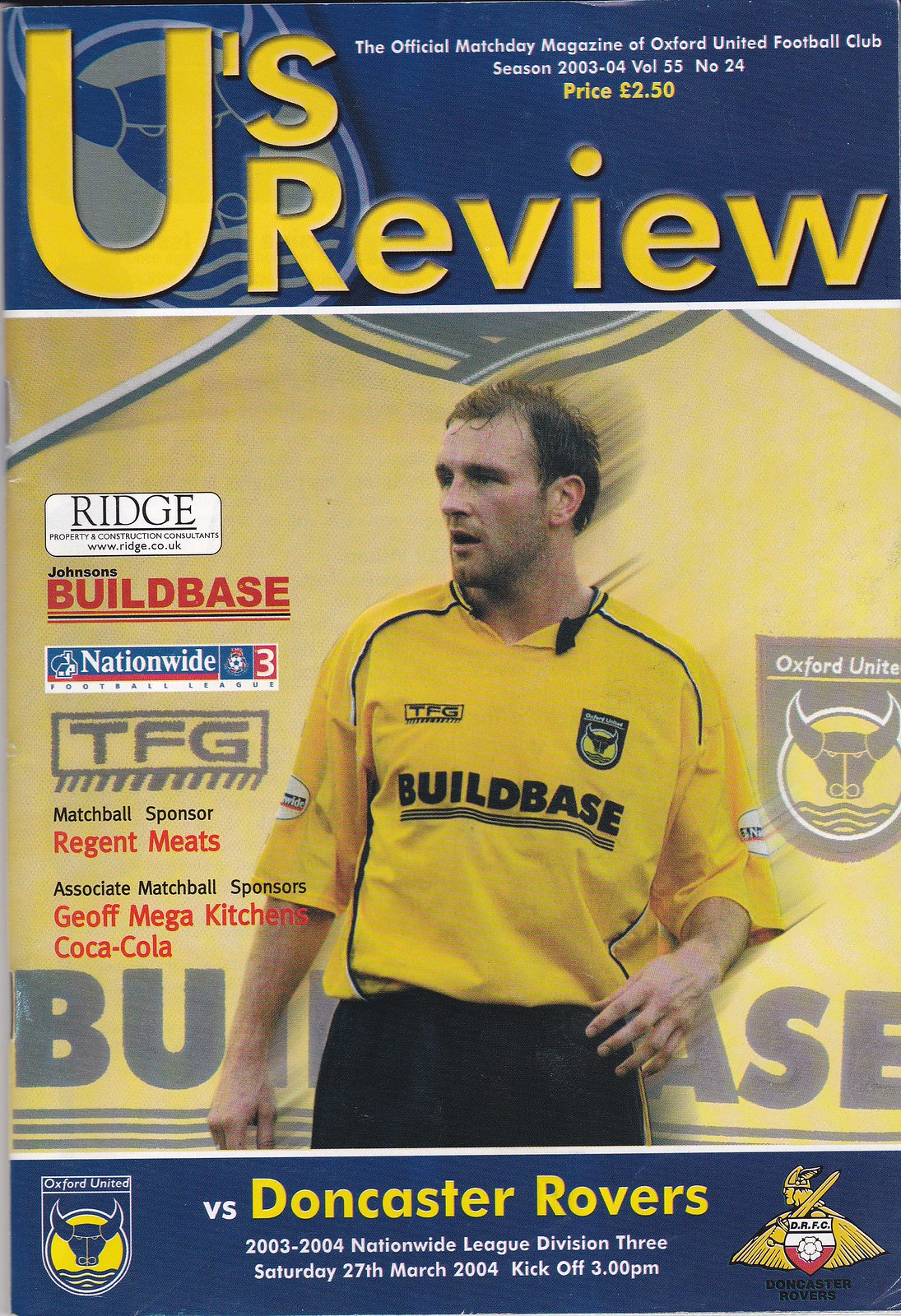This is the official Match Day magazine cover for Oxford United Football Club, Season 2003-2004, Volume 55, Number 24, priced at £2. The top header is navy blue with prominent yellow text reading "U’s Review." Above it, smaller text states: "The Official Match Day Magazine of Oxford United Football Club." The cover features a player in mid-game, wearing the team's Build Base-sponsored yellow jersey. The background is a golden yellow, matching the team's colors and logo. Various sponsor logos including Ridge Property and Construction, Johnson's Build Base, Nationwide, TFG, Regent Meats, Jeff Mega Kitchens, and Coca-Cola are present on the left side. The bottom banner details the match specifics: "Oxford United versus Doncaster Rovers, Nationwide League Division 3, Saturday 27th March 2004, kickoff 3 p.m."